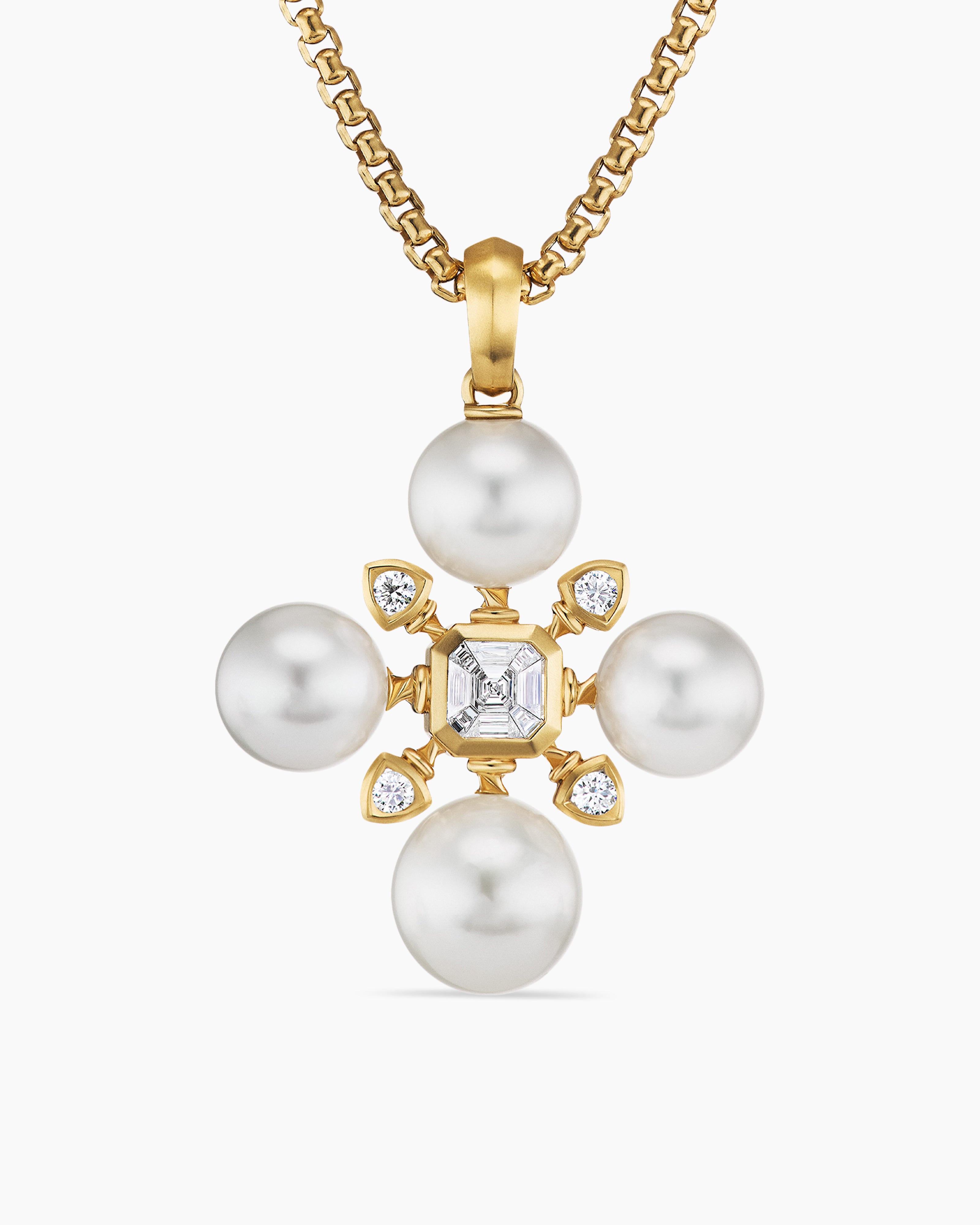The image depicts a highly detailed close-up of an elegant necklace set against a white cream-colored background, with a slight shadow cast by one of the pearls below. The necklace features a gold chain that transitions into an ornate pendant. The pendant consists of four pearls arranged in a cross-like shape, though not joined by lines, surrounding a central cluster of diamonds. In the very center, a prominent square diamond is encased in gold, flanked by four triangular gold settings each holding a small round diamond. The main colors of the necklace are gold and white, contributing to its luxurious and sophisticated appearance.